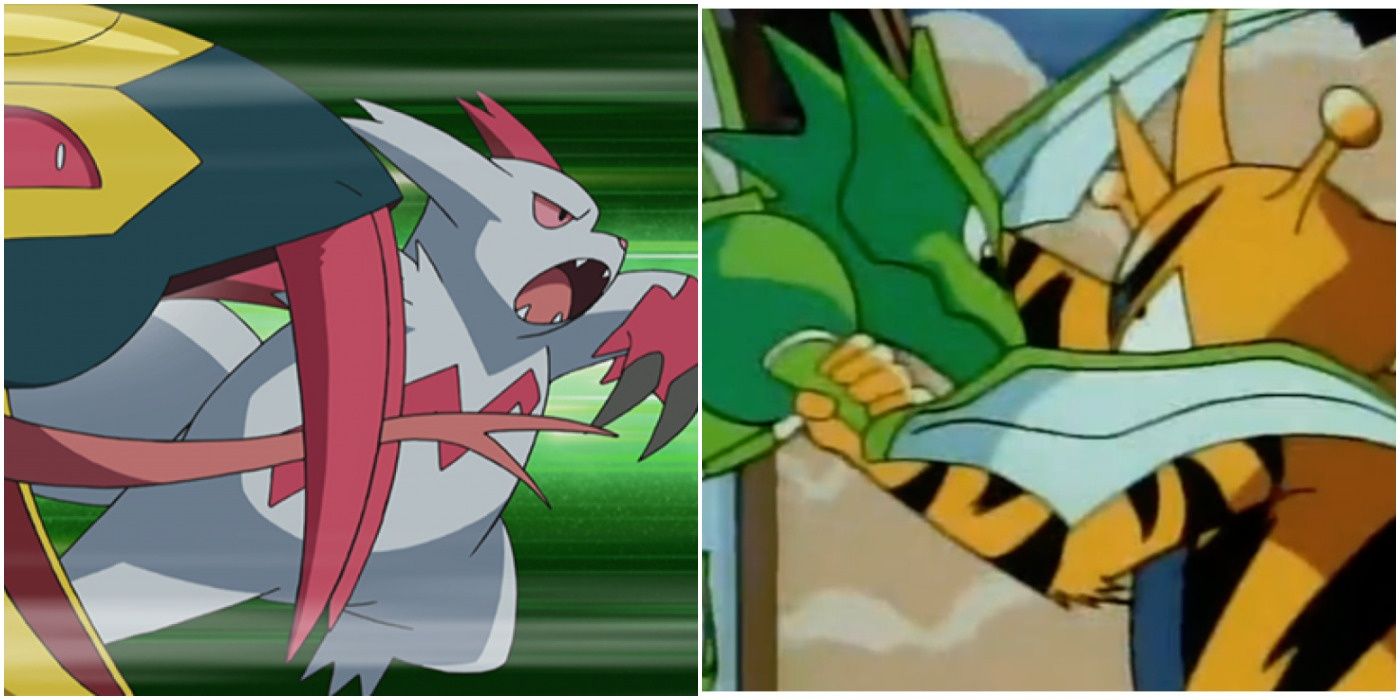This illustration comprises two side-by-side cartoon panels, each depicting fantastical creatures in dynamic poses. The left panel features a white, demonic creature with a pink lightning bolt insignia on its chest, sharp pointed ears, and a set of long claws. Its mouth is open, showing ferocity, and the background streaks with green lines suggest it is moving swiftly to the right. Accompanying this demon-like figure is a snake-like creature with large red fangs, a forked tongue, and a tri-color head — black, yellow, and red.

To the right, the second panel displays a tiger-patterned monster with both horns and antennae-like structures protruding from its head. This creature, which has blue, brown, red, and white stripes, grips a green dragon-like entity by one of its wings. The dragon appears to be snarling back, indicating they are locked in combat. Both panels, showcasing these animated and vividly designed characters, reflect the dramatic tension typical of a children's morning cartoon.